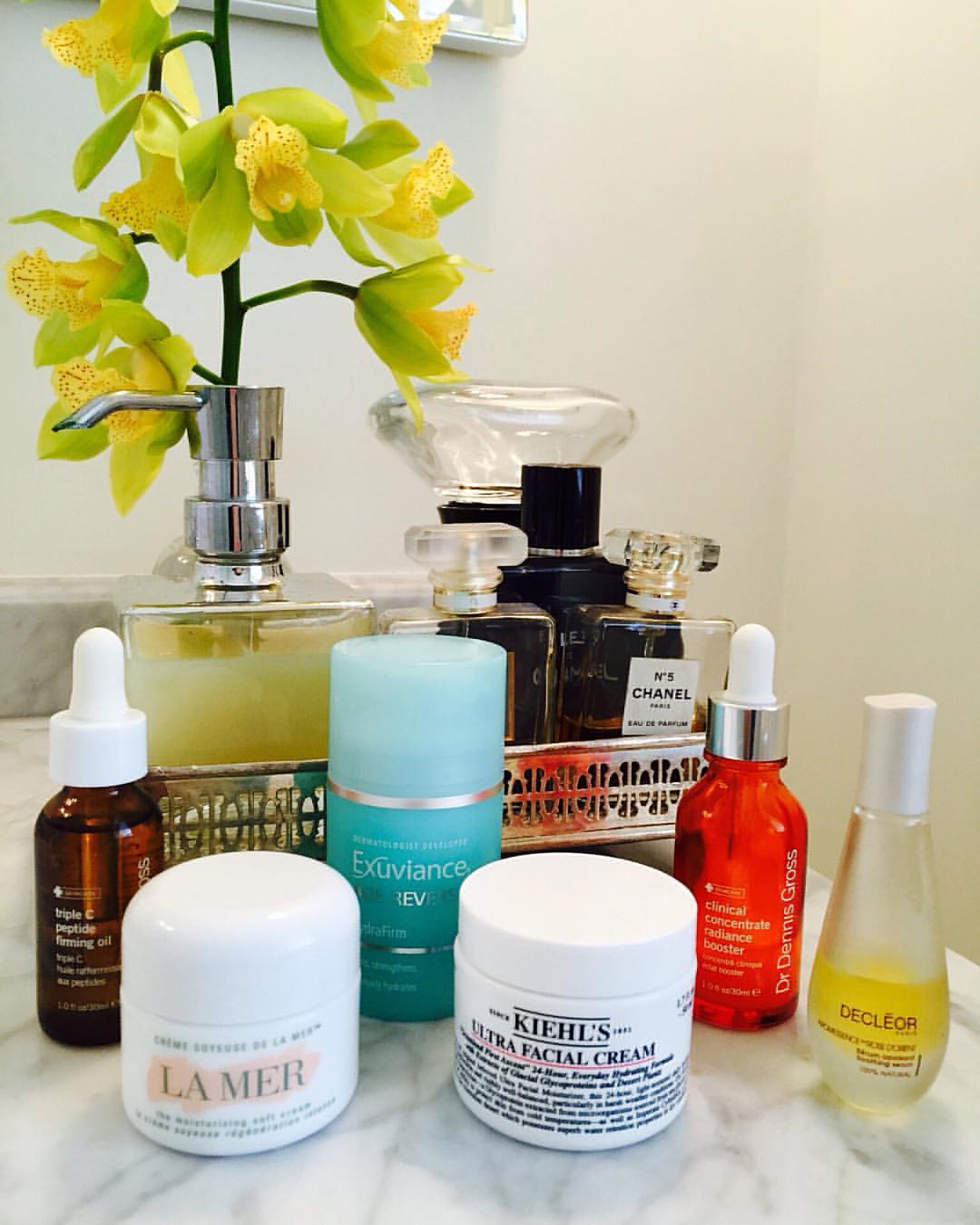A detailed photo taken on a bathroom counter reveals a meticulously arranged collection of personal care items and a decorative touch in the background. The backdrop features a simple white wall and a vibrant plant with yellow-centered and green-bordered flowers, elegantly displayed in a vase. The plant is situated behind a small section containing various fragrances and pumps, accentuating the sophisticated setup. 

Prominently displayed is a silver pump filled with yellow liquid. Nearby, a notable Chanel No. 5 perfume bottle stands out among other black bottles topped with clear plastic caps, though their labels are not discernible. These items reside in a silver basket adorned with a pattern reminiscent of basketball circles.

In the forefront, placed on a pristine white and gray marble counter, are six distinct products arranged diagonally. At the leftmost end, a dropper labeled CCC Peptide Firming Oil is positioned next to a white jar of La Mer cream. Adjacent to these, a taller teal-colored Exuviance product stands, followed by Kiehl's Ultra Facial Cream in a white jar. Moving rightward, a white and silver-top dropper bottle labeled Dr. Dennis Gross Clinical Concentrate Radiance Booster adds a splash of red to the display. Finally, at the furthest right, a bottle of Decléor, featuring yellow and beige hues with a silver-like top, completes the elegant collection.